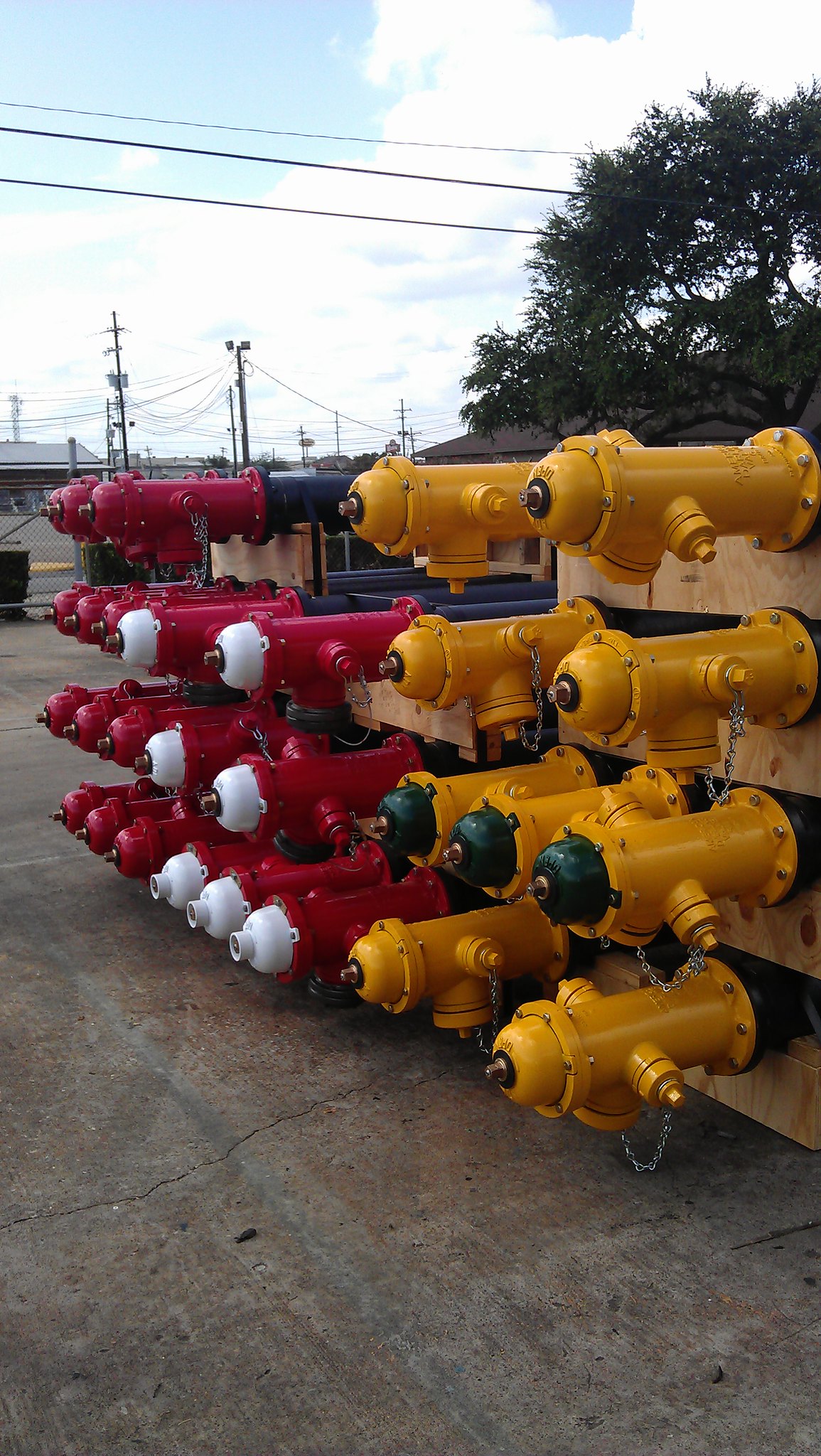In this vibrant outdoor color photograph, a collection of fire hydrants is strikingly displayed, horizontally arranged on wooden pallets or crates. The scene is set on what appears to be a paved concrete pad or possibly a dirt field, with the fire hydrants prominently placed in the foreground. On the left side of the image, a number of all-red fire hydrants are visible, with pipes extending from their backs. Adjacent to these, in the middle section, are more red fire hydrants, some capped with white tops, while others have matching red caps. In the foreground to the right, a series of yellow hydrants catch the eye, with a couple of them sporting dark green caps. The various colors and arrangements create a visually compelling pattern.

The background features the bright blue sky dotted with fluffy white clouds, indicating a very sunny day. Structures such as buildings and utility poles with overhead wires can be seen in the distance, suggesting some industrial activity. Additionally, a large tree with dark green leaves and interspersed branches provides a natural contrast against the man-made elements.